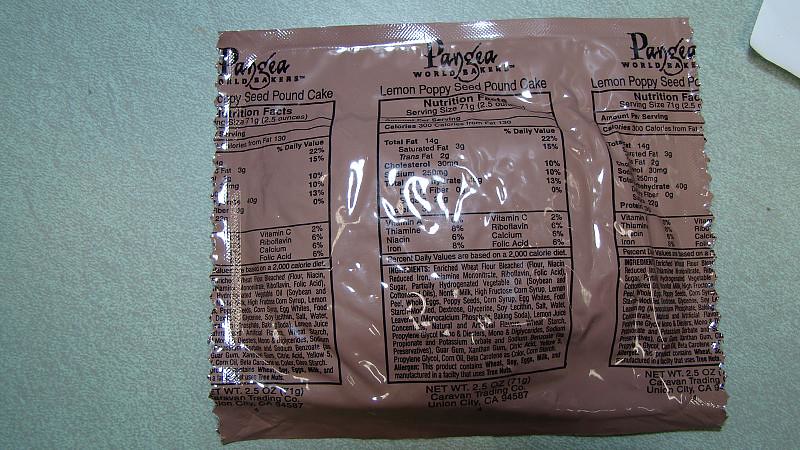The image features a brown MRE (Meal, Ready-to-Eat) packet prominently displayed on what appears to be a green textured surface, possibly a table or floor. The front of the MRE packet is clearly marked with the title "Pangea," indicating that it contains a Lemon Poppy Seed Pound Cake. The packaging reveals the nutrition facts in three different locations, with partial views on the left and right sides, suggesting that the product is mass-produced. This dessert item has a net weight of 2.5 ounces. The nutrition facts are enclosed in black boxes with a brown background, while the text itself is in black font. Additionally, the packaging provides the origin information, stating that the product is distributed by the Caravan Trading Company, located in Linen City, California.